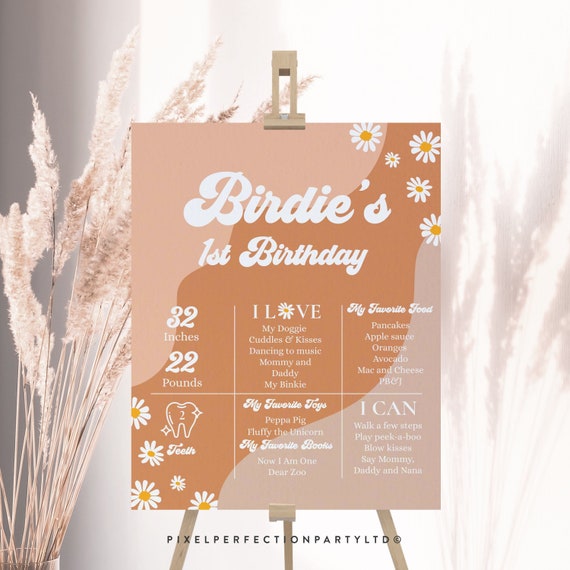The image appears to be an advertisement for an invitation-making company, showcasing their ability to create celebratory signs. The focal point is a sign displayed on a light tan-colored art easel against a pink backdrop adorned with long-stemmed plants and flowers on the left-hand side. The sign, in various shades of beige and orange with white daisies in the corners, declares "Birdie's First Birthday" in an elegant font. The sign is detailed with personal milestones and favorites: "32 inches, 22 pounds. I love my doggie, cuddles and kisses, dancing to music, mommy and daddy, my binky." It lists favorite foods like "pancakes, applesauce, oranges, avocado, mac and cheese" as well as "two teeth," favorite toys "Peppa Pig and Fluffy the Unicorn," and favorite books like "Now I am One, Dear Zoo." Achievements include "I can walk a few steps, play peekaboo, blow kisses, say mommy, daddy, and nana." The bottom of the sign notes "Pixel Perfect on Party Limited ©," indicating the company behind the creation.